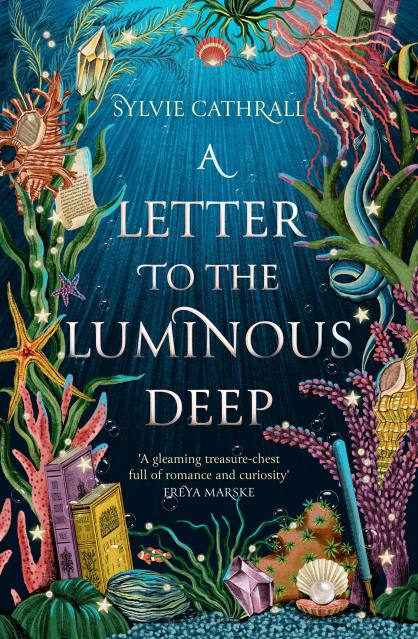The cover of the book "A Letter to the Luminous Deep" by Sylvie Kethrell beautifully combines text and illustration to evoke an underwater ambiance. The top of the cover features the author's name, Sylvie Kethrell, in a clean, striking font. Below it, the title "A Letter to the Luminous Deep" is emblazoned in a white, subtly yellowed text. Directly beneath the title is a quote from Freya Marsk: "A gleaming treasure chest full of romance and curiosity."

The illustration vividly portrays an underwater scene, transitioning from light blue at the top to darker hues as it approaches the ocean floor, mimicking the natural gradient of ocean depths. The scene is teeming with colorful marine life and objects. Various types of algae in purple, green, and pink shades adorn the backdrop, along with starfish in yellow and purple, a white shell with a pearl, and a blue eel. A gleaming crystal is showcased at the upper left corner, while a distinctive blue pen is visible at the lower right. Scattered throughout are books and shelves, suggesting an oceanic library. Jellyfish with pinkish-red hues float near the top, adding an ethereal touch. The entire visual composition frames the central text, creating a captivating and immersive book cover.